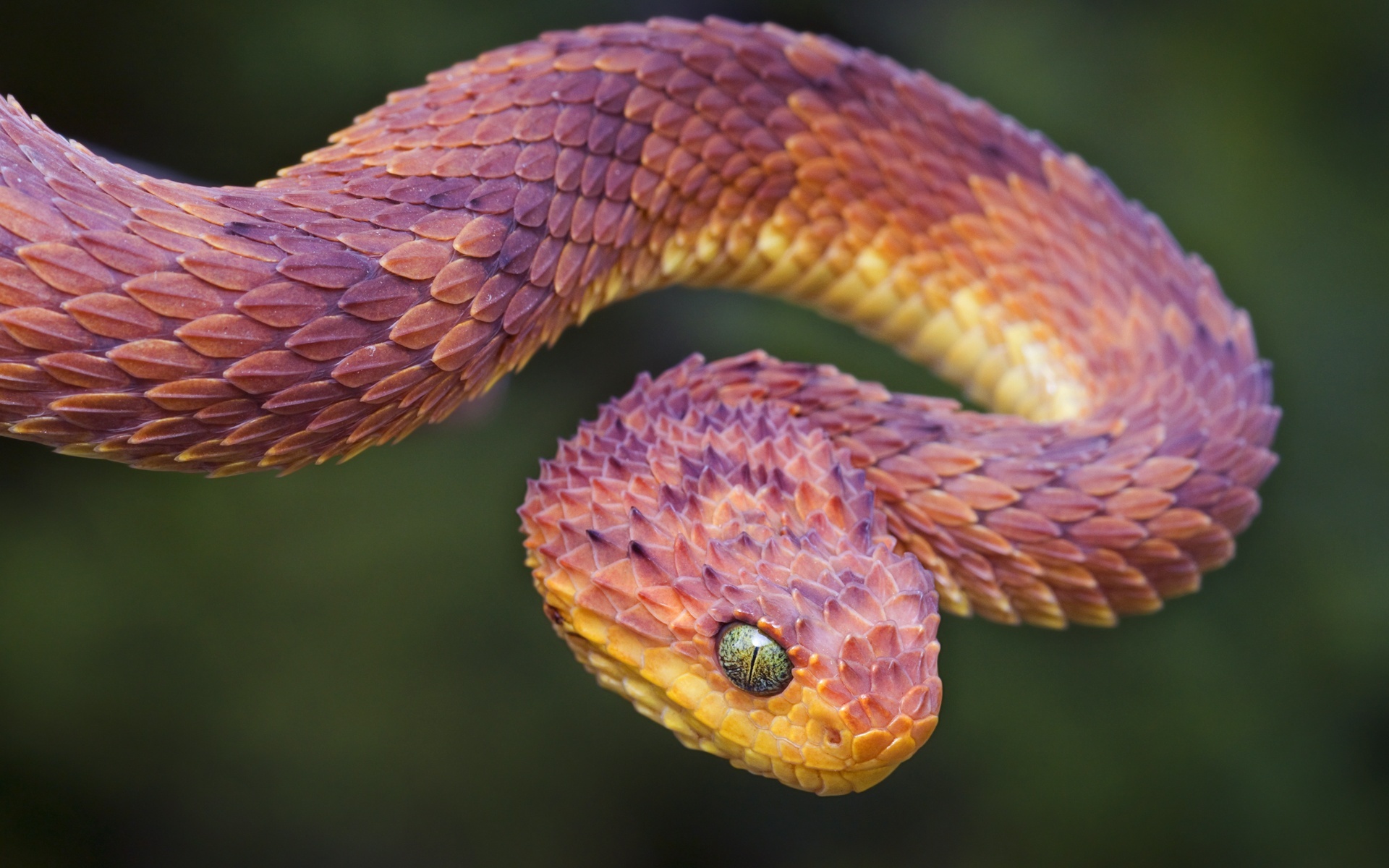This high-quality photograph, reminiscent of a textbook image or a National Geographic feature, showcases a mesmerizing snake against a blurred, deep green background with hints of lighter green and occasional black. The snake is captured in vivid detail, with its scales clearly visible. The picture focuses on the snake's upper body as it emerges from the left side, curves towards the middle, and then turns dramatically. The head, closer to the viewer, features striking green and yellow eyes with a black slit for the pupil, giving it a dragon-like appearance. The snake's face and mouth are highlighted by yellow hues, while its body displays a stunning palette of fiery tones—ranging from purple and yellow to orange and red. The scales, resembling the overlapping tips of pine cones or almonds, add to the snake's captivating beauty.